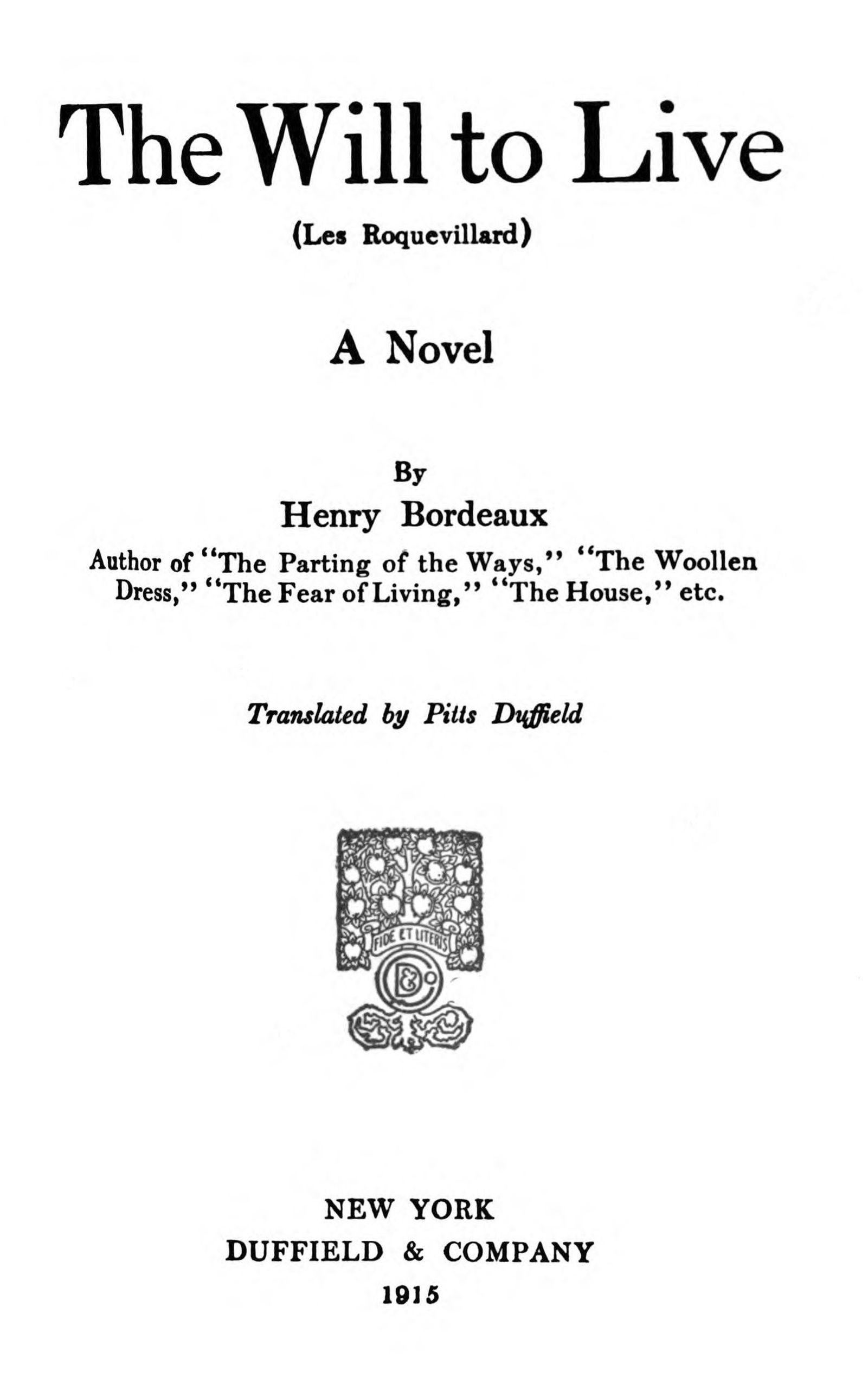The image appears to be the title page of a book presented on a white background with black text. At the top, in bold black letters, it reads "THE WILL TO LIVE." Below this, in parentheses, it states, "LES ROQUEVILLARD," which is the original French title. The text continues to describe it as "A novel by Henry Bordeaux," with Bordeaux being the author of several other works including "The Parting of the Ways," "The Woolen Dress," "The Fear of Living," and "The House," among others. This is followed by "Translated by Pitts Duffield." 

Centered on the page is the publishing company's insignia, which includes the text "FIDE ET LITERIS" on a banner adorned with floral designs above and twisted lines below. Finally, at the bottom of the page, it mentions "New York, Duffield and Company, 1915." This logo features a decorative, possibly tree-like symbol inside a square, adding a touch of artistry to the otherwise text-focused page.